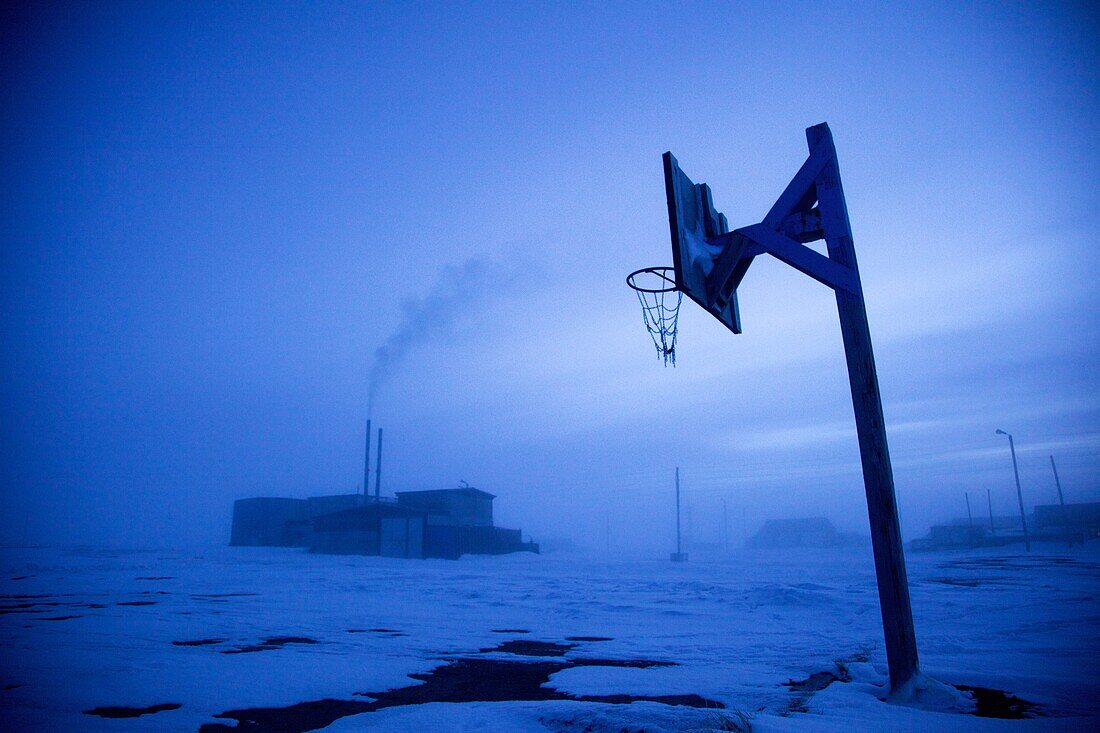The image portrays an eerie, desolate winter scene bathed in a dim blue light, resembling an arctic or Siberian landscape. The ground is covered in snow, emphasizing the cold, bleak atmosphere. In the foreground stands a homemade basketball hoop, crafted from scrap wood and tilting slightly, with a forlorn chain net that is partially missing. This poignant detail contributes to the sense of abandonment and poverty. Far behind the hoop, several large buildings are faintly visible, some featuring tall smokestacks, with one emitting smoke or steam. Additional structures and distant light poles further suggest an industrial yet remote setting. The overall composition, coupled with the blue tint, enhances the image's haunting, almost otherworldly quality.